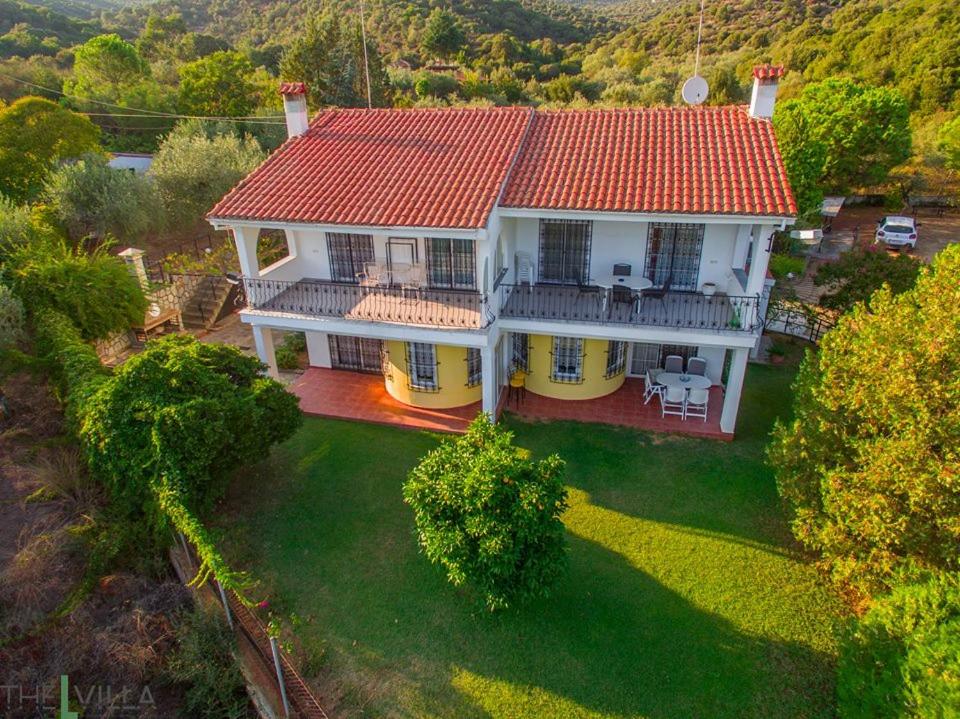This aerial photo, likely taken by a drone, captures a serene, outdoor landscape in a horizontal layout, showcasing the lush, green backyard of a well-maintained two-story house surrounded by dense forestry. The house, centrally positioned, features a distinctive red shingled roof and white walls accented with yellow paint on the lower level. Its architectural charm is highlighted by two identical segments, each with its own balcony. The upper balconies are furnished with tables and contrasting chairs—white on the right side and blue on the left—while the lower level has a white round table with several chairs only on the right side. 

The green grass and the numerous trees around the property enhance its picturesque setting, with large trees prominently positioned on the left, middle, and right sections of the yard. A small white car is parked on the right, adding to the scene's everyday warmth. 

In the lower left corner, a bit of overgrown vegetation and dead plants is visible, contrasting the neatly kept lawn. This corner also displays a logo reading "The L Villa," with "The" and "Villa" in grey and 'L' in green. Bounding the property is a fence with some areas overgrown with weeds, beyond which the dense forest begins. This image captures a beautiful, tranquil home nestled in a flourishing green environment.